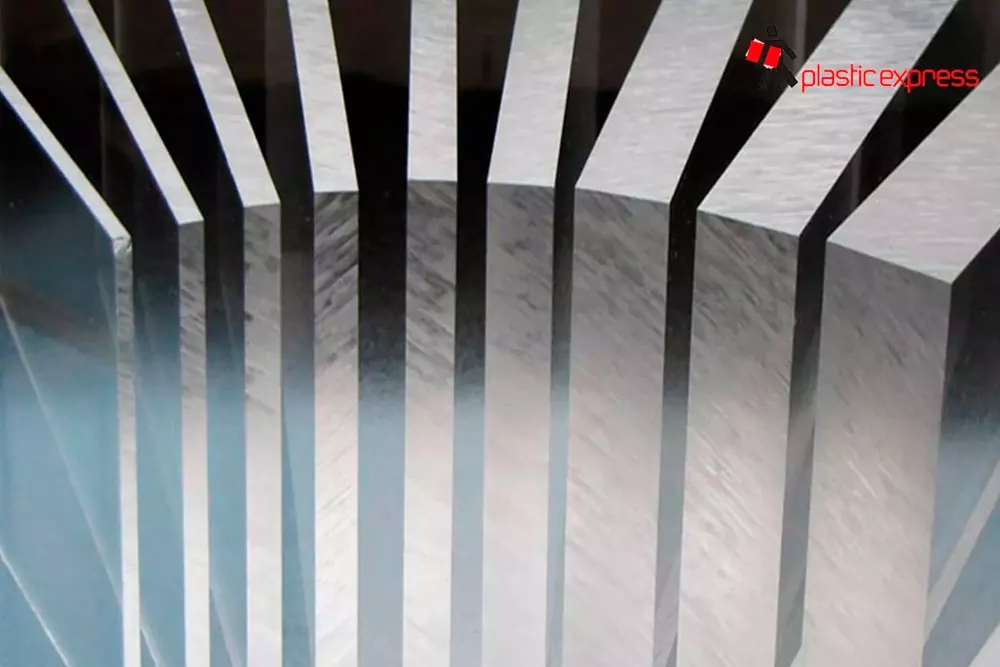The image showcases an acrylic or plastic sheet adorned with black vertical stripes centrally located, which transition to horizontal stripes as they extend towards the ceiling. The background features a grayish-brown hue with a marble-like or grainy texture, giving it a sophisticated appearance. The ceiling shares a similar grayish coloration. There's a light source on the left side, creating a gradient effect across the sheet, which adds a blurry glow, making it appear lighter as it ascends compared to the ceiling. The photograph also contains text in the top right corner that reads "Plastic Express" in red. Overall, the interplay of light and dark grays, combined with the textured background and prominent black stripes, creates a dynamic and visually intriguing composition.